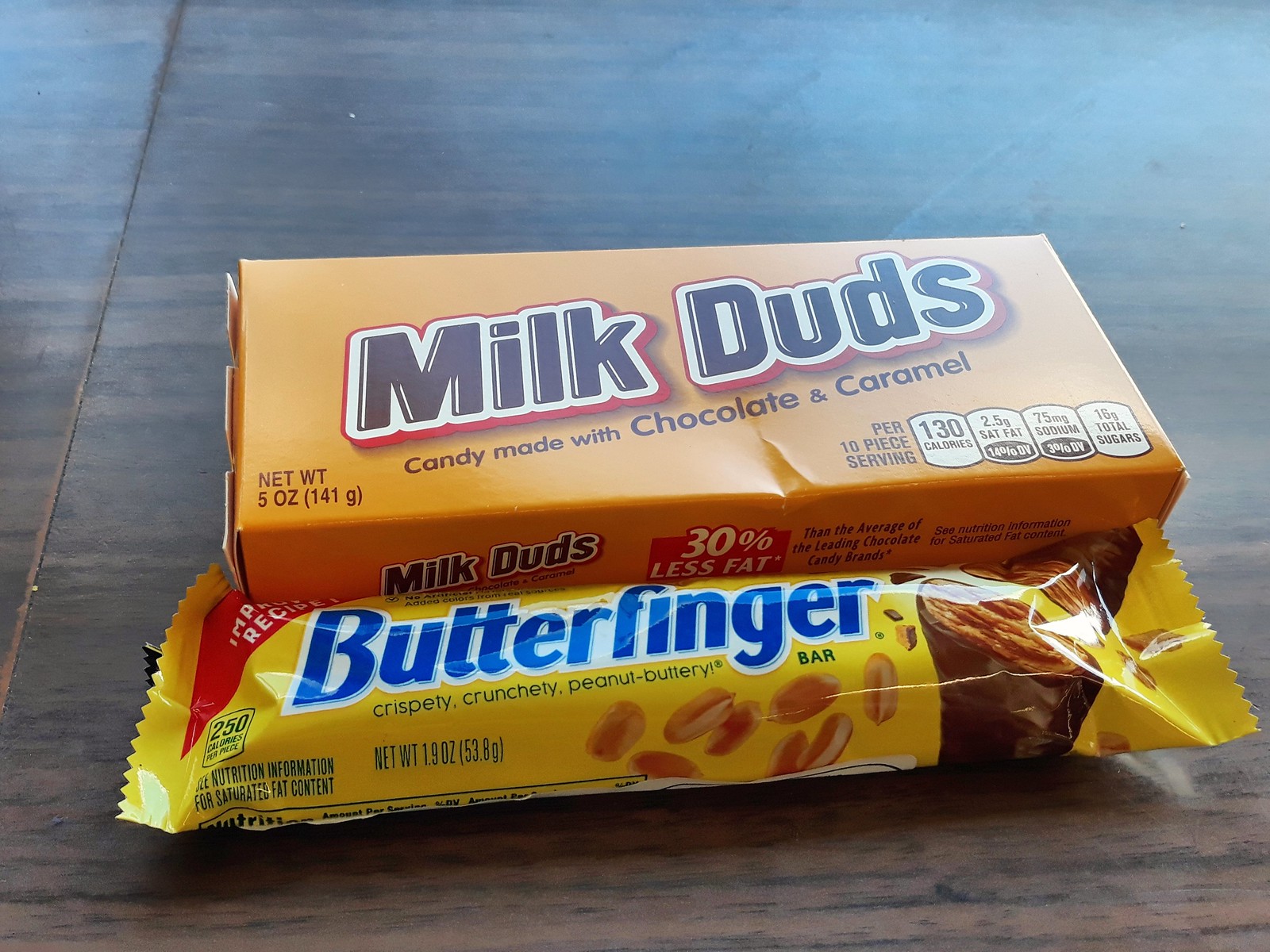In the image, a wooden tabletop with distinctive black grains and a visible seam running down the middle hosts two candy items. The first item is a rectangular, orange-yellow box of Milk Duds, featuring brown letters outlined in white that read "Milk Duds." The box prominently states that the candy is "made with chocolate and caramel" and includes detailed nutritional information such as “130 calories, 2.5g saturated fat, 75mg of sodium, and 16g total sugars” for a 10-piece, 5-ounce (141 grams) serving. Directly beneath the Milk Duds box lies a yellow-wrapped Butterfinger candy bar, slightly angled up against it. The Butterfinger wrapper is adorned with blue text outlined in white, along with a red triangle in the top left corner proclaiming an "Improved Recipe." The wrapper also highlights the bar's texture and flavor with the words "Crispity, Crunchity, Peanut Buttery Bar" and displays an illustration of the bar, revealing its rich brown exterior and light honey brown interior with peanuts scattered around. Both candies are sealed, their packaging intact.